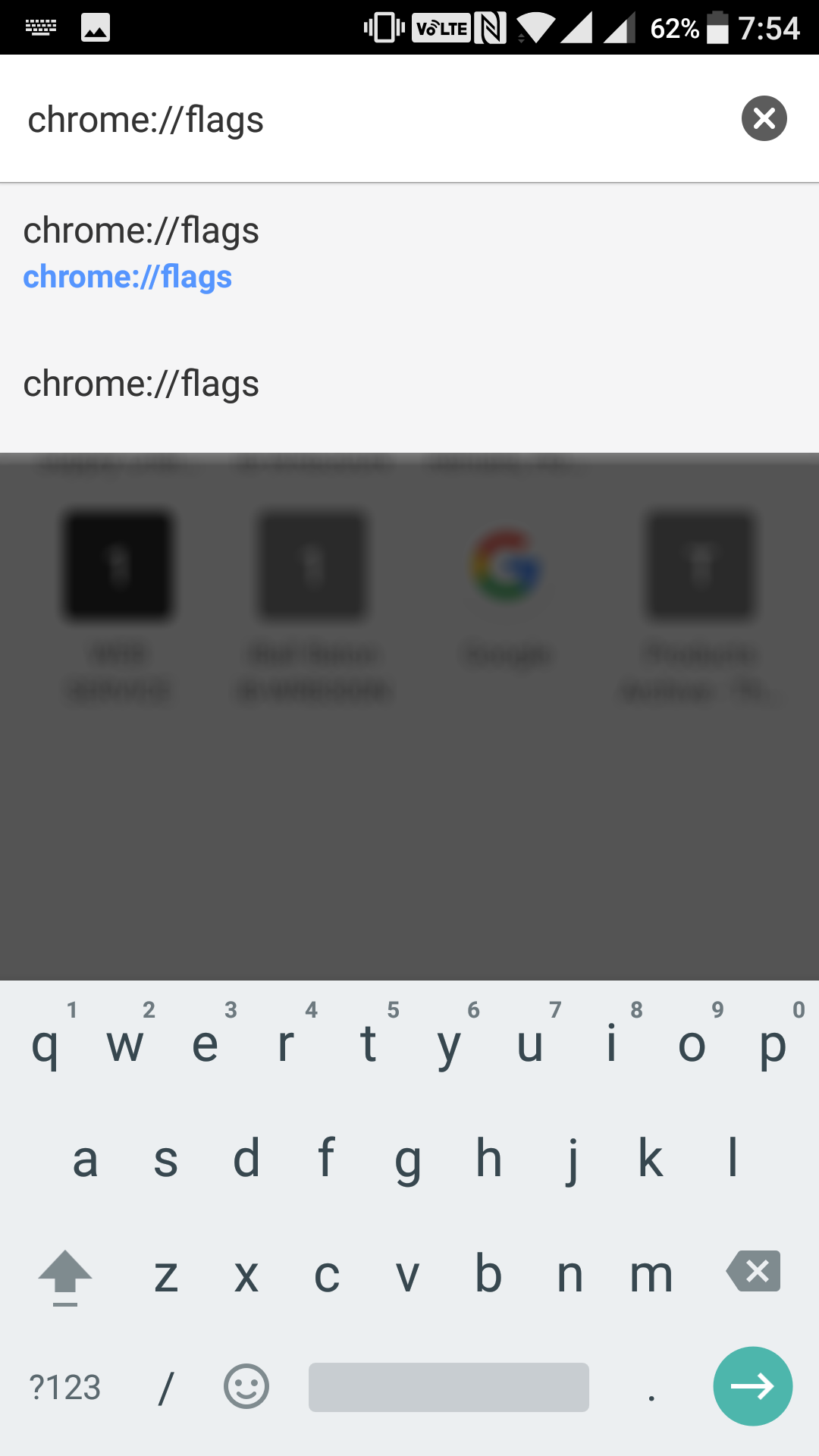A screenshot depicting the Chrome "flags" settings page is visible. The URL "chrome://flags" is prominently displayed multiple times at the top, emphasized in blue. The screen indicates 62% completion with a reading of "754" and an 'X' button for exiting the view. Below this, another "chrome://flags" URL appears, signifying the same settings page is being shown.

A gray rectangle overlays part of the screen, suggesting a section with numerous apps beneath it. Below the gray area, a virtual keyboard is shown, featuring the standard layout. The keyboard includes:

- Numeric keys (1-0) at the top.
- Alphabetic keys in the middle.
- On the left side, an up arrow for capitalizing letters.
- A "1, 2, 3" button which would switch from letters to numbers.
- Special character keys including a slash and a smiley face for emoji access.
- A space bar at the bottom.
- On the right side, an 'X' button presumably to close the keyboard.
- A green circle with a white arrow pointing to the right, likely to submit or enter the data typed.

The detailed layout of settings and the keyboard indicates a typical configuration and navigation process within the Chrome browser on a mobile or touch device.